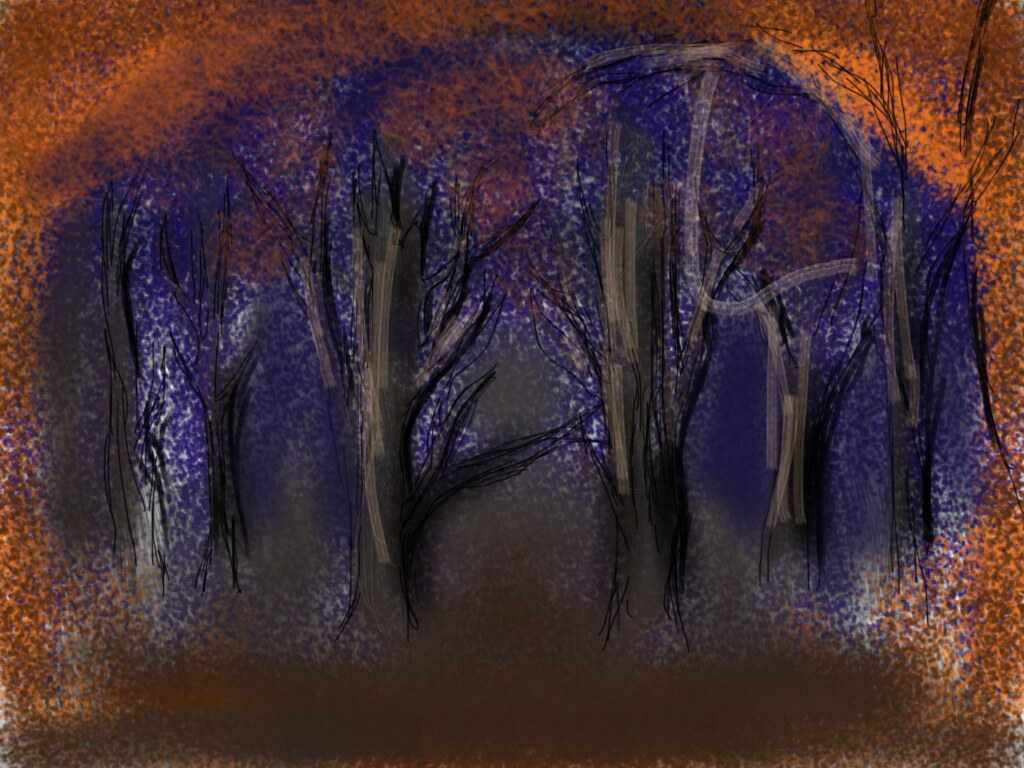The image is a dark, abstract digital sketch of barren trees. Approximately five or six bare tree trunks with sharp, rough lines dominate the center, giving a haunting feel. They are sparsely colored with rough shades of brown, mimicking light and shadow. Surrounding the trees is a textured, speckled effect with an arch of orange dots and a central area of purple dots, creating a distinct contrast. The ground beneath the trees is a more solid dark brown, differing from the speckled texture above. This artwork's impressionistic style evokes a mysterious, possibly spooky forest scene, with layered dots adding to its depth and complexity.